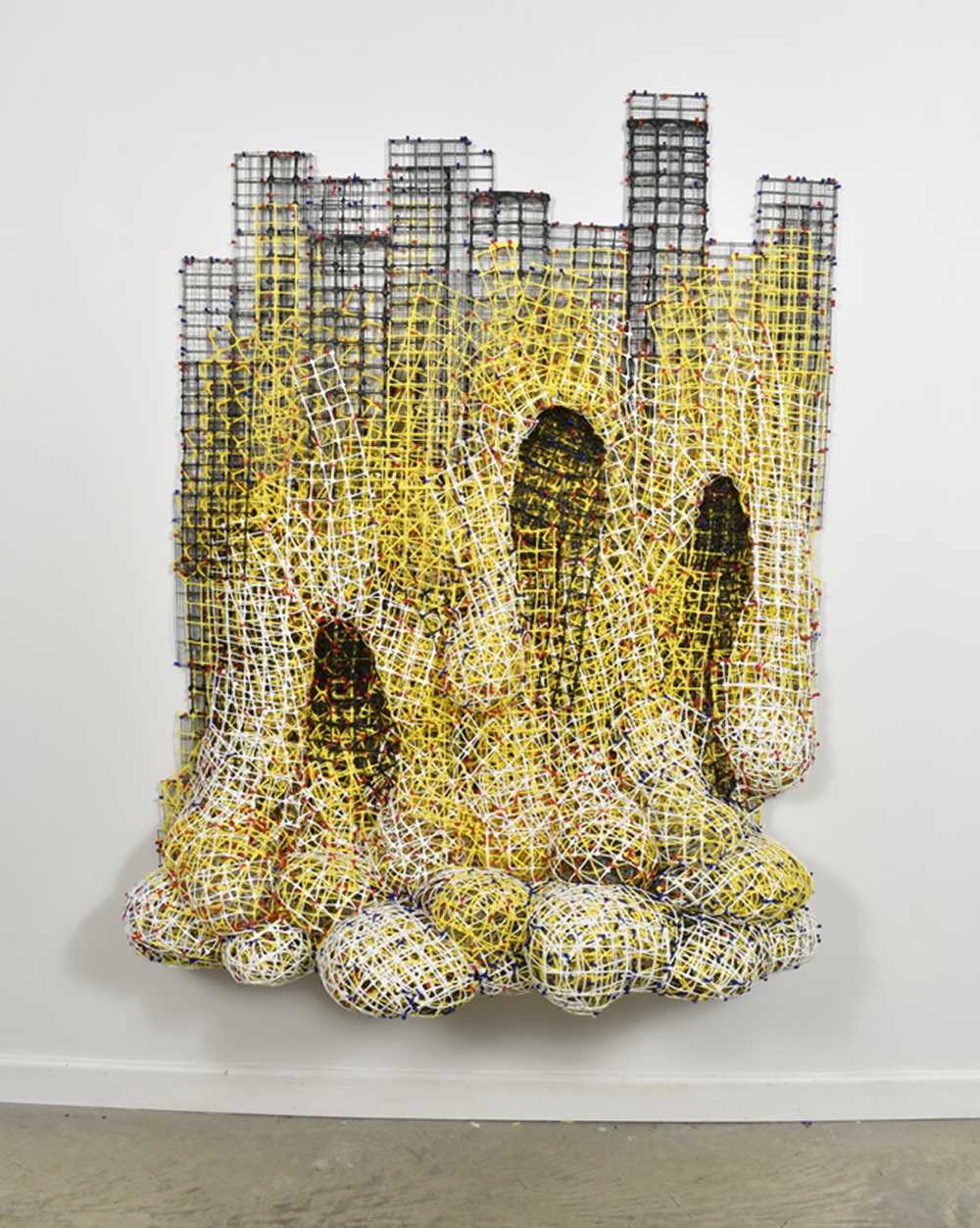This horizontal rectangular image showcases an intricate piece of handmade artwork mounted on a white wall. The artwork is composed of a wire mesh structure featuring black and yellow hues, creating an abstract and visually striking composition. The mesh forms appear to suggest tall towers or tree trunks, with some sections covered in green yarn-like material to indicate plant life. At the base of the towers, the mesh descends into several round balls, also crafted from the same material. These balls rest on a background that transitions from a brown color at the very bottom, resembling a skinny baseboard, to a white surface. The overall effect is that of a complex yet elegant wireframe landscape that is both modern and organic, capturing the viewer's attention with its unique blend of materials and colors.